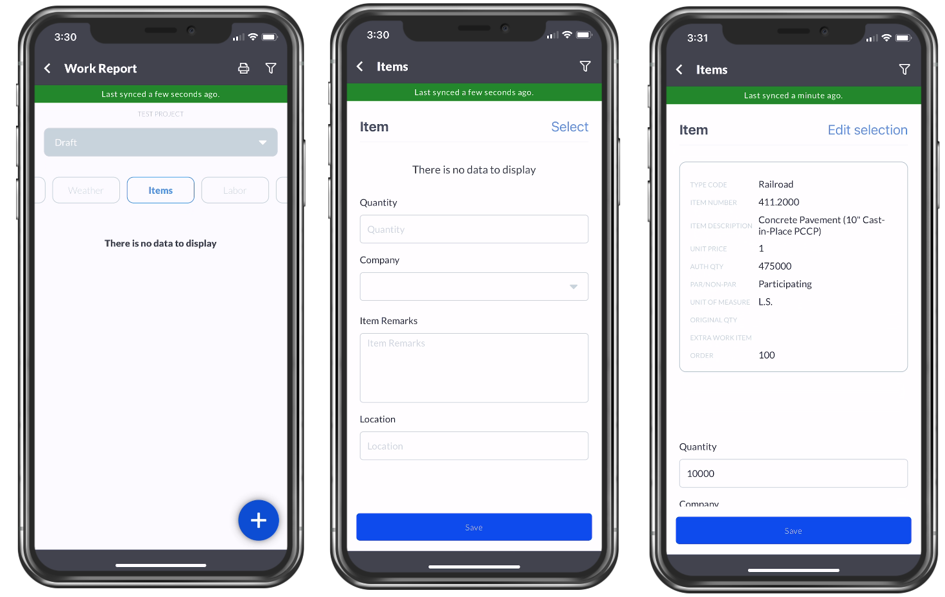In this image, three iPhone screens are displayed horizontally side by side. Each screen features an interface with a gray title bar at the top. The two screens on the left and center display the time as 3:30, while the screen on the far right shows 3:31. In the top-left corner under the time, each screen has a back arrow; the first screen labels this section as "Work Report," whereas the other two are labeled "Items."

Below the title bars, there is a green synchronization status bar on each screen. The left and center screens show "Last synced a few seconds ago," while the right screen indicates "Last synced a minute ago."

The first screen shows the text "Test Project" in gray on a white background. Below that, there is a light gray, rounded-rectangle box stretching across the screen, labeled "Draft" in white text with a downward arrow on the right side. Beneath this, there are three equally rounded boxes; the left and right box text is unclear, while the middle box, highlighted by a blue border, reads "Items." Further down, black text on a white background states "There is no data to display." At the bottom of the screen, a blue circle with a white plus sign is present.

The center screen also displays "Items" in the top-left corner under the green bar, followed below by a blue-highlighted "Select" option. The screen reads "There is no data to display" in black text on a white background. Accompanying this are label fields for "Quantity," "Company," "Item Remarks," and "Location."

On the far right screen, under the green bar, "Items" is displayed again in the top-left corner, followed by the option "Edit Selection" in blue. Unlike the other screens, this one has all fields filled in, but the specific details are not legible.